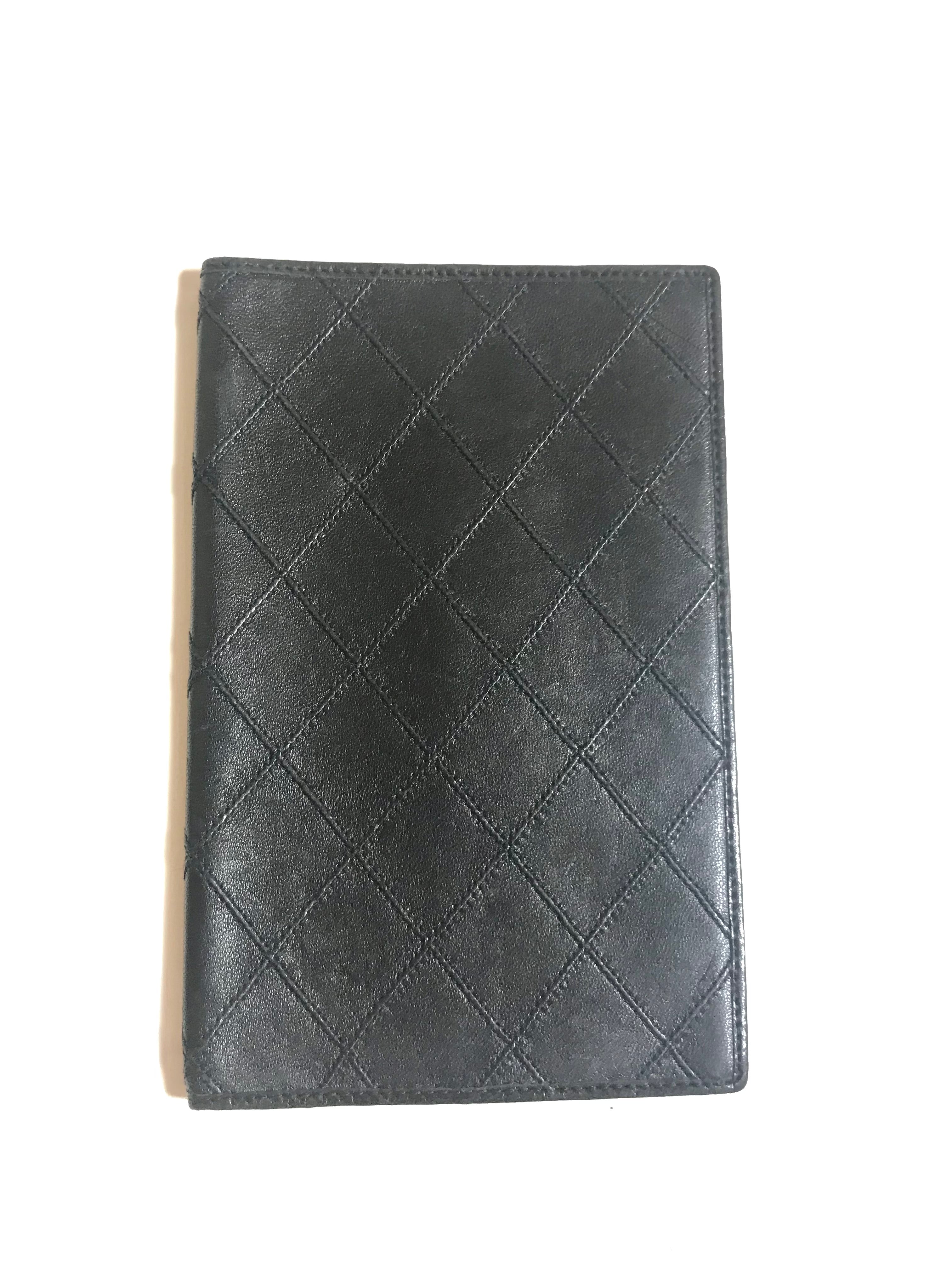This is a close-up, color photograph depicting a leather-bound book, potentially a diary, journal, or planner. The object is set against a solid white background, allowing the details of the book to stand out prominently. The book features a dark, almost black leather cover adorned with an intricate herringbone pattern created by diagonal stitching, forming diamond or square shapes across the surface. This stitching is embossed, giving it a textured feel that one could easily discern by touch. The book is visibly smaller than an 8.5 by 11 sheet of paper and does not display any title, words, or numbers on its cover. The image is well-lit with natural lighting, providing clear visibility of the book's detailed craftsmanship.